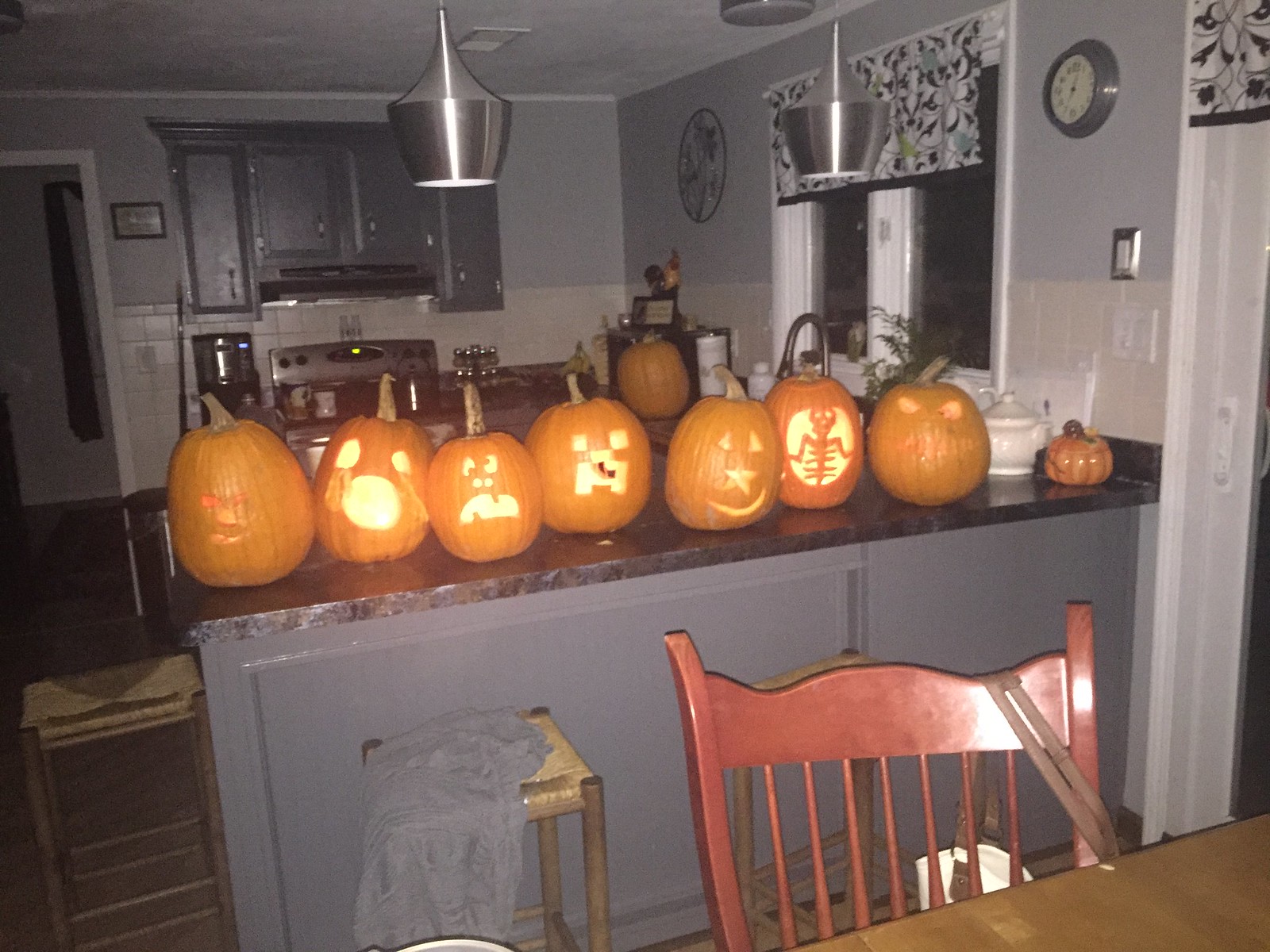The photograph captures an interior view looking from a dimly lit dining area into a kitchen, which is illuminated by the camera flash. The dining table, partly visible in the foreground, is accompanied by a wood chair draped with a bag. A peninsula-style counter extends from the right side of the kitchen to divide the space, adorned with nine pumpkins—eight of them in a horizontal row across the nearly black marble countertop, and one small porcelain pumpkin off to the right. The pumpkins display various intricate carvings; some depict faces—ranging from scary to surprised, frowning, and even one with a star-shaped nose—while another features a skeletal image. Intriguingly, five of these jack-o'-lanterns are lit up from within, casting a bright, warm glow that highlights their designs. Additionally, an uncarved real pumpkin can be seen on another counter in the background.

The kitchen's dark gray walls and lower cabinet sides complement the counter's darker hue. Two backless stools sit at the counter, one adorned with a gray scarf. Above the counter, two lights hang, providing additional illumination. The scene is framed by gray cupboards above a visible stove, and a clock and a curtained window above the sink further accentuate the backdrop.